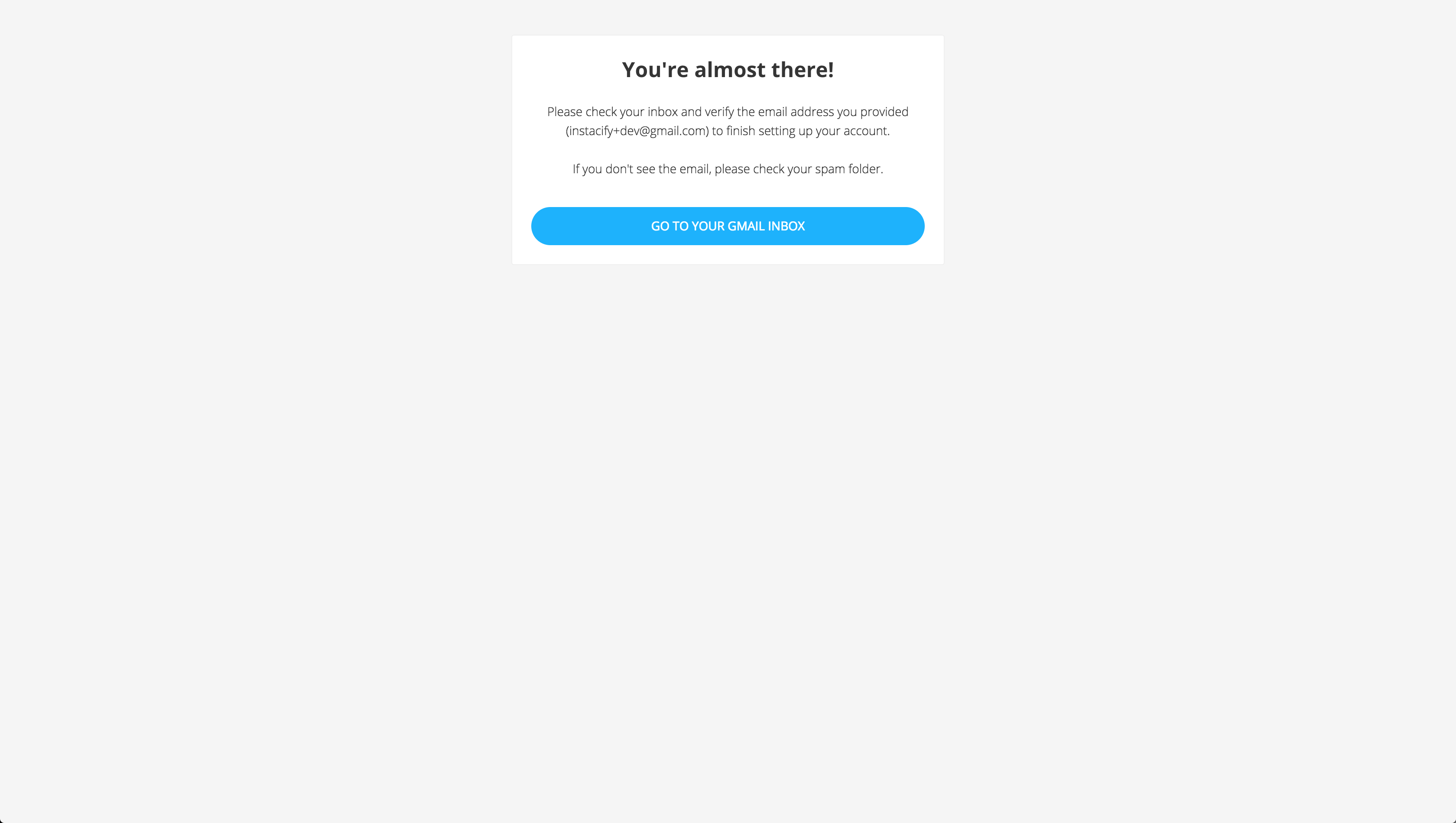The image features a grey background, predominantly simple and unobtrusive. Centered towards the top is a prominent white dialogue box. At the upper portion of this dialogue box, in bold black text, it reads: "You’re almost there!" followed by an exclamation mark. Below this, in a much smaller font, the text guides the user to check their inbox and verify the email address provided, which is explicitly listed within the message.

The message reads:

"Please check your inbox and verify the email address you provided to finish setting up your account. If you don’t see the email, please check your spam folder."

Beneath this informative text, there is a large, wide blue button with rounded corners. The button is designed for easy interaction and clearly marked as actionable, directing users to their Gmail inbox with a simple click. This setup is indicative of an email confirmation process, likely part of setting up a new Gmail account or reactivating access to an existing one. This security measure ensures that the person attempting to gain access is the rightful owner of the email address, thereby preventing unauthorized access.